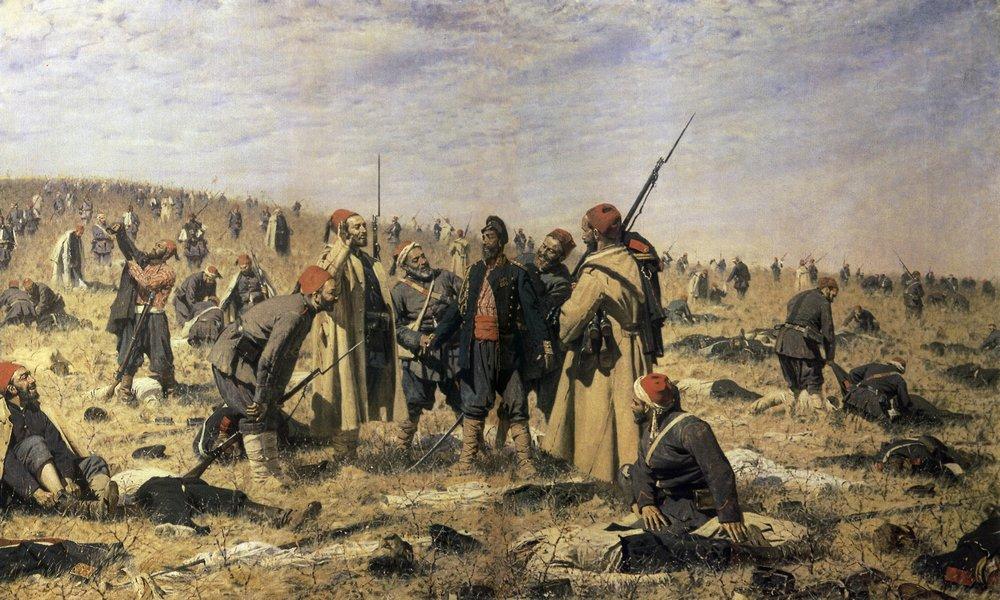The painting is a detailed depiction of the aftermath of a battle. It features a vast, sandy-colored grassy field littered with the bodies of many fallen soldiers, likely numbering in the hundreds. In the foreground, there is a group of about six to eight men, possibly leaders, standing and conversing—perhaps discussing the recent battle or preparing for another. These men are notable for their distinctive attire, wearing red caps, some identifiable as fezes, along with light brown coats. Their weapons include rifles with bayonets, suggesting a historical setting that might be around the World War I era, though with a Middle Eastern flair given the dress and equipment. The sky above is covered in serious, gray clouds, casting a somber and overcast light on the scene. The composition is horizontal, with the group of standing men slightly to the left of the center and the horizon line centering the image.